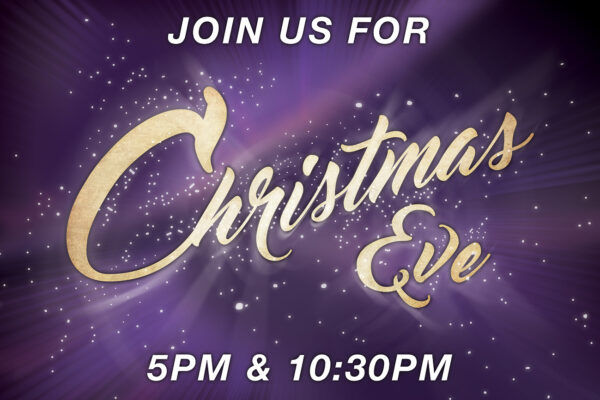The image features a nuanced, purple background with a celestial feel, adorned with white dots resembling stars. At the top, bold white text in all caps reads, "JOIN US FOR." Centered in the middle, large, elegant, gold cursive letters spell out "Christmas Eve." At the bottom, the event times, "5PM and 10:30PM," are displayed in white, all-caps text. The overall design suggests that this is an invitation or advertisement, likely a flyer or poster, encouraging attendance at a special Christmas Eve event.